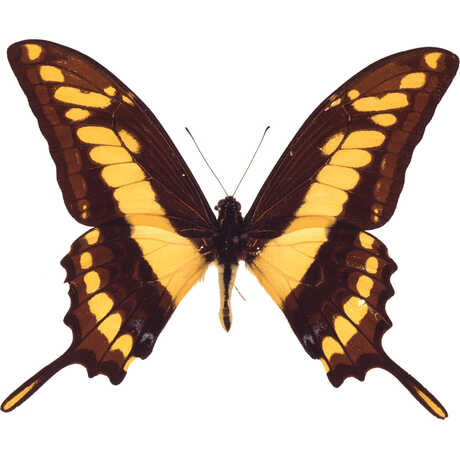The photograph captures a striking butterfly with its wings spread open against a plain white background, making the delicate details of the insect highly visible. The butterfly features large, symmetrical wings that exhibit a captivating pattern of dark brown outlined edges with golden yellow and orange hues. The intricate design includes speckled yellow circles and scalloped lower wings, each with two elongated projections extending outward. The butterfly's body is adorned with contrasting colors: a dark, nearly black center with a bright yellow edge, and a notable yellow stripe down its middle. Its thin, brown antennae stretch upwards in a graceful V-shape. The overall symmetry and vivid coloration evoke comparisons to a monarch butterfly, albeit with lighter, more golden tones.